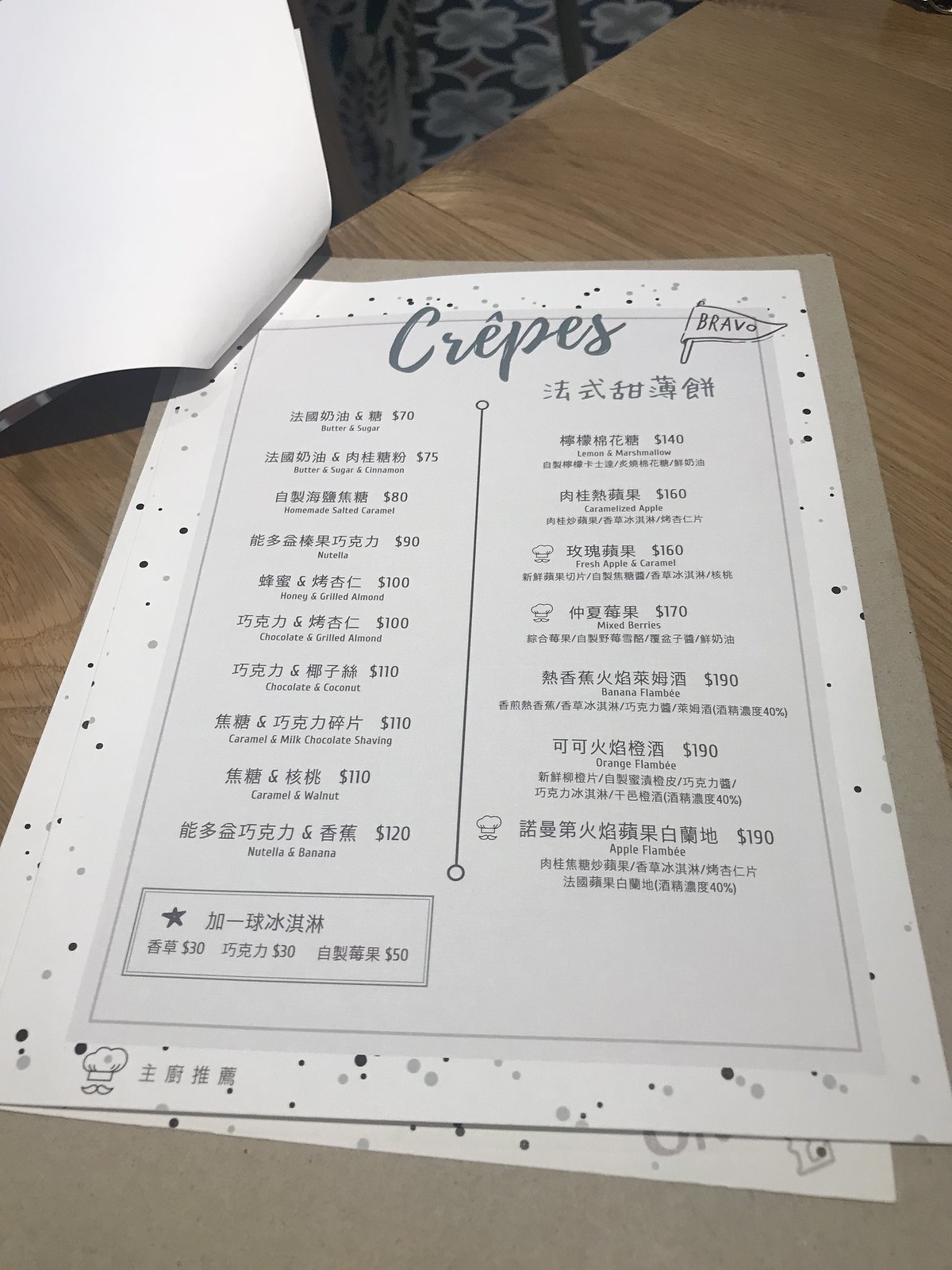This vertically oriented color photograph showcases a menu meticulously laid flat on a wooden table. Dominating the top left corner, the menu is flipped over, revealing its white paper adorned with a delicate pattern of dark gray, light gray, and black speckles – reminiscent of a polka dot effect. Detailed and aesthetically pleasing, the speckled design serves as a border for the menu's content. The crepe-focused menu, titled in a stylish cursive font with "Crepes" at the top, features an illustrated flag labeled "Bravo" to its right.

The menu, centrally positioned but slightly tilted to the right, displays text predominantly in an Asian language, possibly Japanese, Chinese, Korean, or another East Asian script. Divided into two columns by a thin line with decorative circles at both ends, the menu lists various items with accompanying English translations beneath each description. Additionally, a small box located to the left of the left column contains more text, potentially including prices. Beneath the speckled paper, a piece of cardboard provides a sturdy backing, emphasizing the neat presentation of the menu.